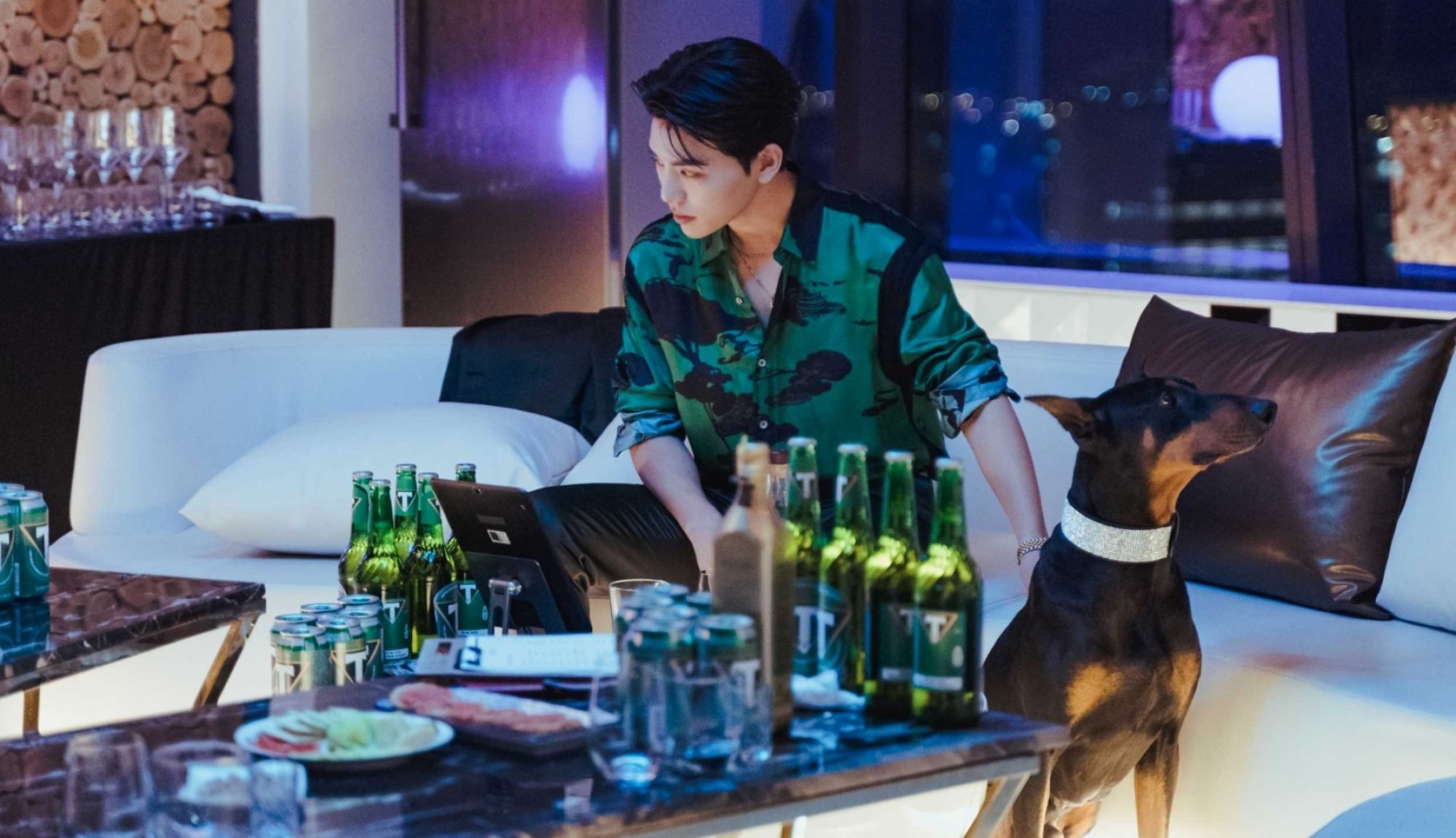The photograph captures a chic, modern living room within a high-floor urban apartment, accentuated by a large window that reveals a dazzling night-time cityscape. At the center of the image sits a young Asian man on a pristine white leather couch adorned with black and white pillows. The man, dressed in an attractive green silk shirt with sleeves rolled up and black silky pants, sports a gold bracelet or watch on his left wrist and has his black shiny hair slicked back and parted in the middle.

The man is looking towards the left side of the image, while at his left side, his loyal Doberman Pinscher dog with a white collar gazes eastward, in the opposite direction. He rests his left hand on the dog’s back. The table before them has a marble top and is cluttered with unopened green beer bottles and glasses, suggesting preparations for an imminent gathering. Additionally, there are five more beer bottles on the floor beside the table. Plates of food, including one with sliced tomatoes and cucumbers and another with rolled-up cold cuts, are also present on the table. On the left side of the living room, there's a bar area with lined-up wine glasses, further enhancing the sense of an impending festive occasion.